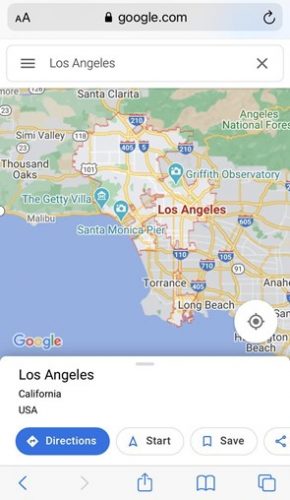Captured on a smartphone screen, this image displays a Google.com search result for "Los Angeles." Dominating the screen is a detailed map of Los Angeles, with "Los Angeles" prominently labeled in red at the center. The map is dotted with various pins marking key locations, such as the Santa Monica Pier, the Getty Villa, the Griffith Observatory, Angeles National Forest, Santa Clarita, Thousand Oaks, Simi Valley, Long Beach, and Hamilton Beach. Yellow roadways and a vast, adjacent ocean are also visible, adding geographic context. At the bottom left of the map, the Google logo is apparent. Below the map, a section reads "LOS ANGELES," followed by "California" and "USA" in capital letters. There are also interactive buttons for "Directions," "Start," "Save," and additional options, providing further functionality to the map.